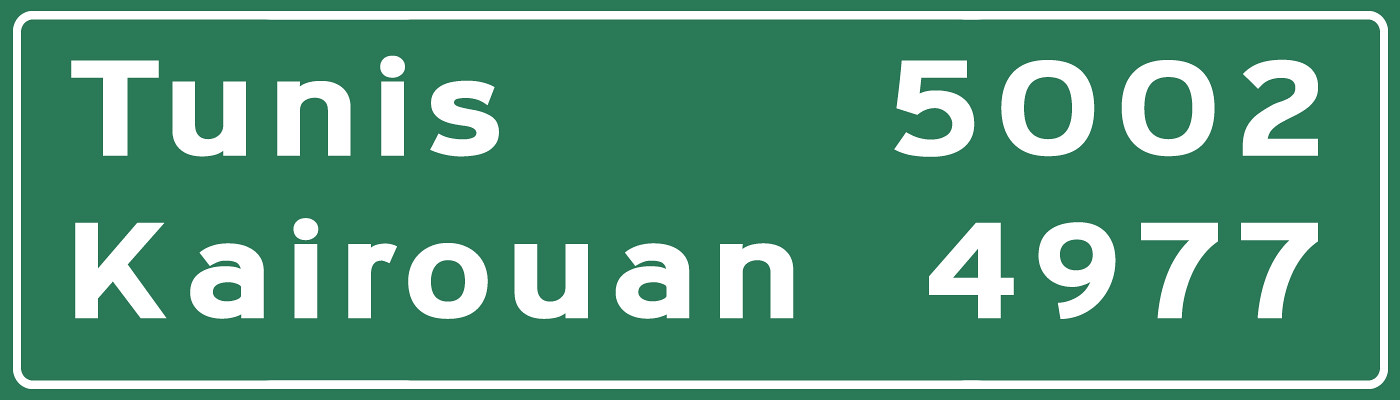This image depicts a rectangular green highway sign with a distinctive white border. The sign dominates the entire photo, measuring approximately 8 inches in length. The upper left section of the sign displays "T-U-N-I-S" in bold white text, accompanied by the number "5002" positioned a couple of inches to the right. Directly below, the sign reads "K-A-I-R-O-U-A-N," also in bold white text, with the corresponding number "4977" similarly styled and located a couple of inches to the right. The sign's text and numbering are prominent, suggesting the distances to these locations, likely in miles. The overall feel is that of an evergreen green typical of highway signage designed to guide travelers.